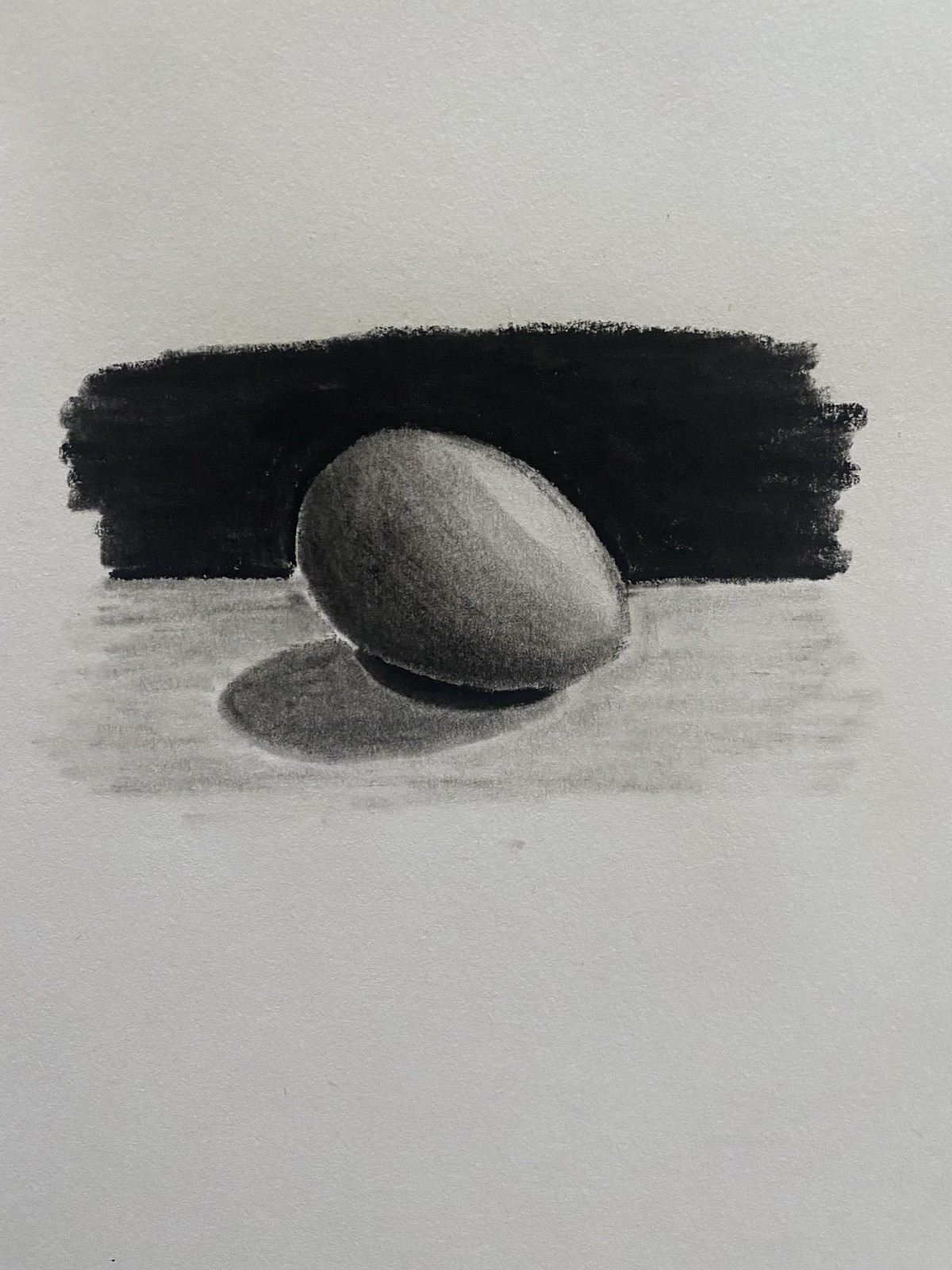A meticulously detailed pencil and charcoal drawing is depicted on white paper, showcasing an egg as the central subject. The egg, with its top pointed down to the right, boasts a symmetrical form and exhibits intricate shading. The left corner of the egg features darker tones that gradually lighten towards the right side. Beneath the egg lies a distinct, dark shadow, while a softer, lighter shadow extends to the lower left. The egg rests on a subtly textured surface, lightly penciled to suggest depth. In contrast, the background behind the egg is densely shaded in a deep black, creating a rectangular shape with uneven edges. This dark backdrop, which includes a defined horizon line that curves up and around the egg, serves to sharply differentiate the egg from its surroundings.